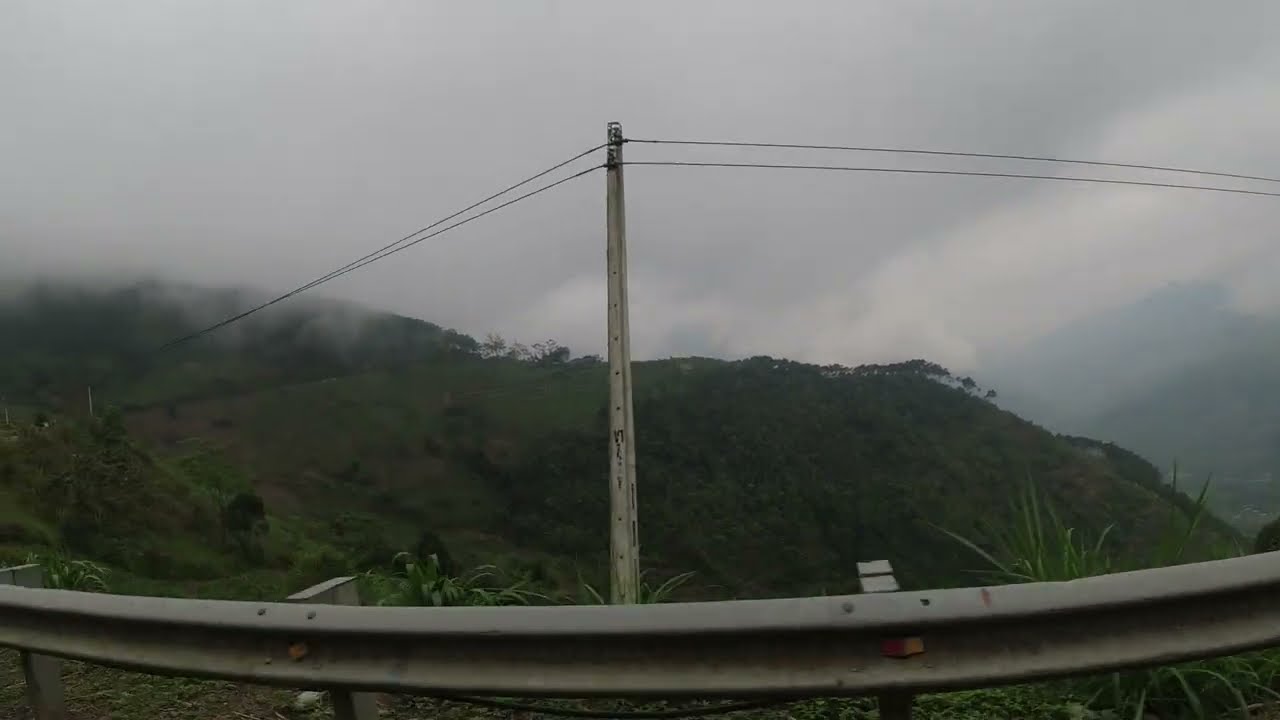The image captures a scenic view from the side of a mountain road, featuring a prominent silver guardrail stretching across the bottom. The guardrail, made of metal and painted gray, lines the edge of the road and prevents vehicles from veering off into the hillside. In the midground stands a telephone pole with wires extending horizontally across the scene, likely in shades of silver or dark gray. Behind the guardrail and pole, lush green hills covered in vibrant grass, shrubs, and trees spread out into the distance. The sky above is heavily overcast, casting a grayish tone over the entire landscape, with dense clouds almost completely obscuring any blue. There's a hint of fog, especially noticeable on the left side and in the distant hills to the right. The road itself appears to loop around in the distance, suggesting a winding path through this mountainous area. This scenic overlook offers a hazy view of adjacent mountains across a valley, enhancing the picturesque but misty atmosphere of the setting.